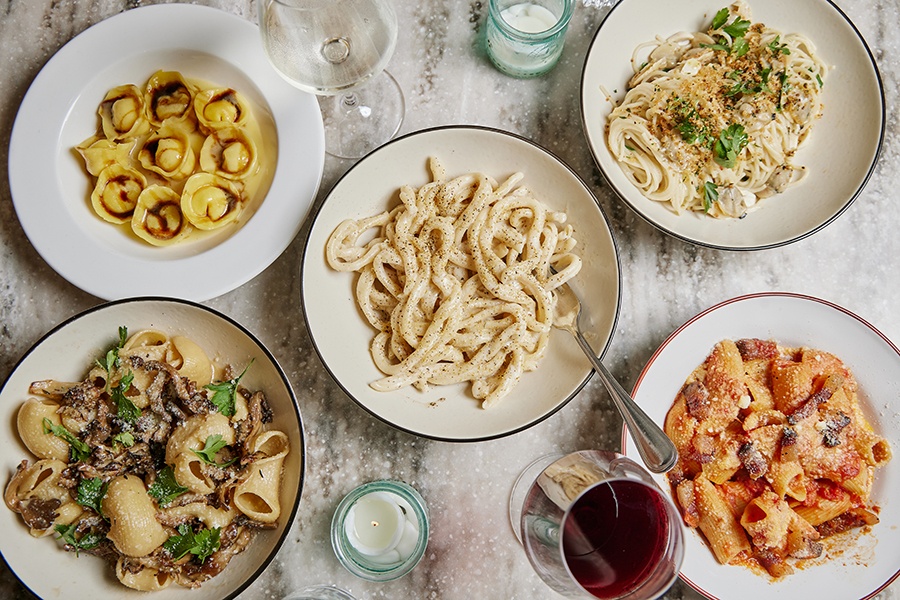This photograph captures an overhead view of five plates of Italian cuisine arranged on a marble-topped table. The central focus is a white, round dish containing thick white noodles coated in a white sauce, with a few pepper flakes sprinkled over them. The plate in the top left looks more like a bowl within a plate and contains open-faced clams or oysters topped with a yellow sauce. Moving diagonally to the top right, there is a plate of thinner, heavily piled noodles garnished with green herbs and a sprinkling of red spice. Directly beneath this, in the lower right corner, is a plate of pasta in a rich red sauce with both red and brown meatballs, and a topping of white cheese. To the bottom left, there is a dish featuring thick beige noodles with bits of brown meat, green herbs, and a sprinkle of white cheese. Beside this plate sits a stemmed glass containing red wine. Complementing the arrangement are two small, clear glass candle holders with lit white candles, one positioned just below and to the left of the central plate, and the other above and slightly to the right. The entire scene is set against the elegant backdrop of a predominantly white marble table with black shading and cloud-like patterns, suggesting a high-end dining experience, likely intended to promote an Italian restaurant, catering service, or a fine dining cookbook.